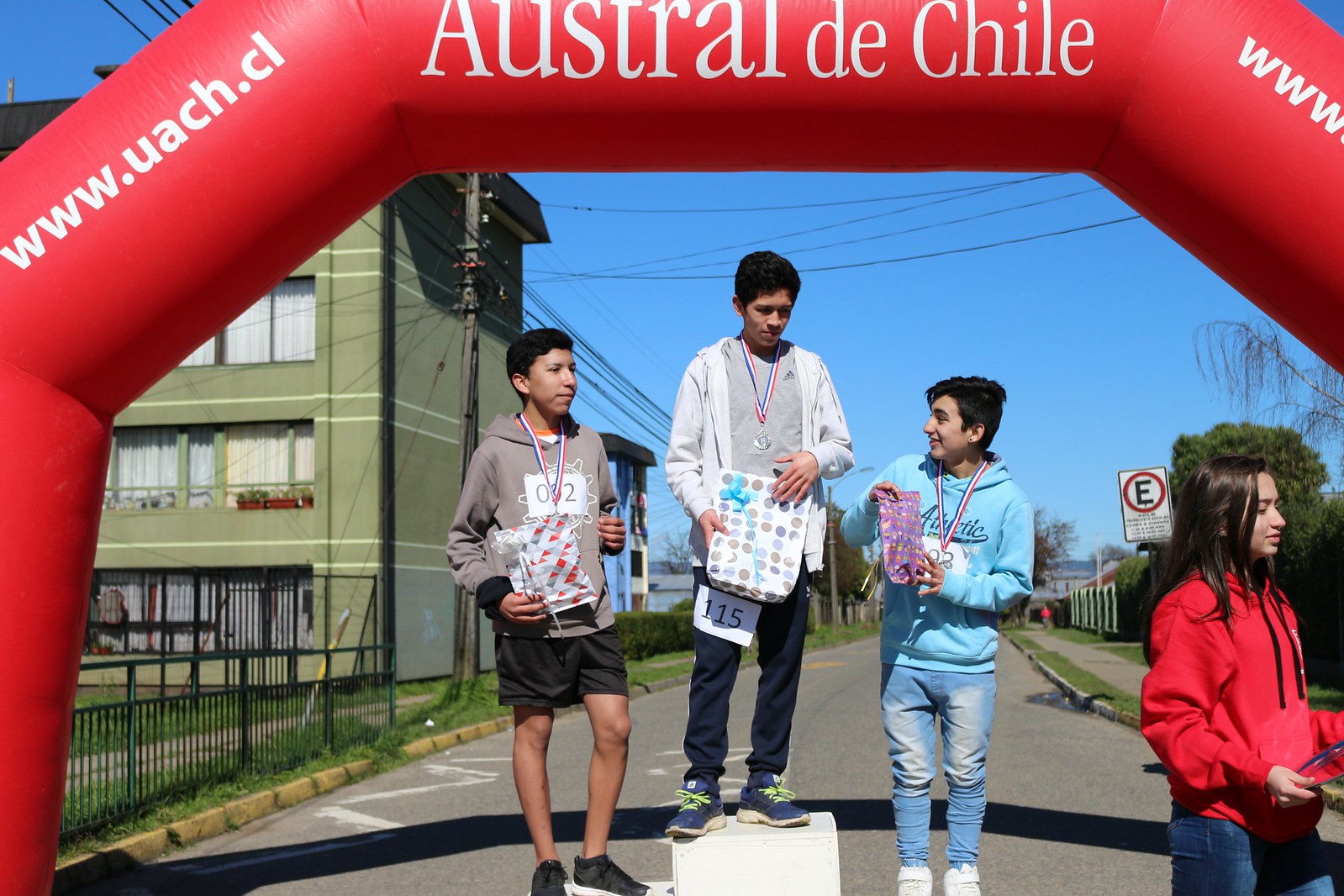In a wide rectangular image, three boys stand on podium blocks after a race, each wearing different colored medals, signifying first, second, and third place. Center stage, the boy on the highest block has black hair, dons a white hoodie with a gray shirt underneath, and a number tag "115" on his leg. Flanking him, the boy to the left, in black shorts and a brown shirt, holds a medal and appears to clutch something. On the right, the third boy, in a blue Aeropostale shirt and blue jeans, holds a pink item. Above them arches an inflatable rainbow-shaped red balloon inscribed "Austral de Chile" and the event’s URL, "www.uach.cl." In the background, on the left, there's a large multi-story light green apartment building next to a gray road bordered by green grass and a sidewalk. To the right, another sidewalk runs along a series of green hedges. Adding to the setting, the sky is blue and the daylight brightens the scene. Off to the right, a girl with long black hair, wearing a red long-sleeve top and blue jeans, appears to be deep in conversation.